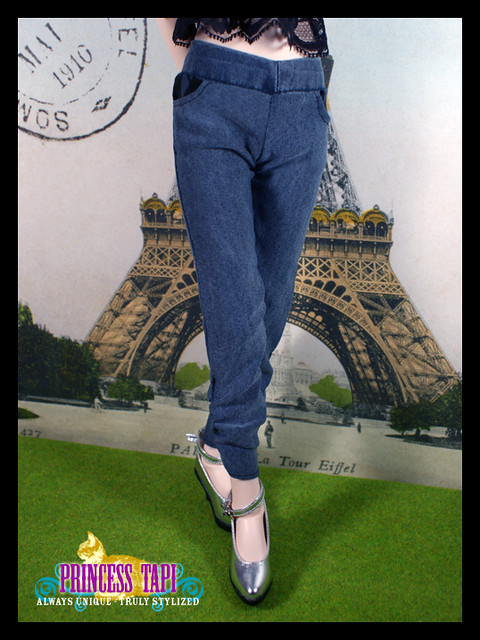This full-color photograph, possibly a postcard, features a woman standing from the waist down in denim soft pants and silver high heels, with her upper half partially visible in a black lace top. She is positioned on artificial grass, and the backdrop is a painting of the Eiffel Tower, complete with a vintage-style stamp that reads "May 1910" near her waist. The image is bordered by a black frame. In the bottom left corner, a gold logo displays an orange cat with the text "Princess Tappy, always unique, truly stylized."